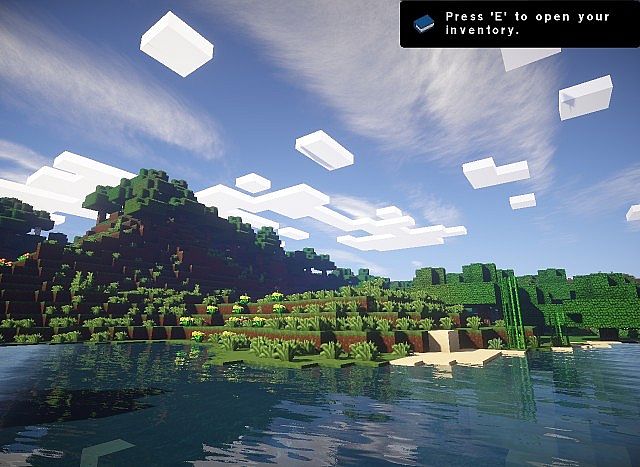The image showcases a seemingly enhanced or modded version of Minecraft with its characteristic voxel-style graphics. The water surface is notably reflective, capturing the bluish hues and mirroring the surrounding foliage with remarkable clarity. The plant life and dirt remain distinctly blocky, while exhibiting bright, vibrant greens that contrast with the detailed water. The skybox is a mix of bright blue, thin white clouds, and the classic blocky clouds, creating an intriguing blend that gives a semi-realistic touch to the traditional Minecraft scenery. In the upper right-hand corner, there is a blue book icon within a black box, displaying the prompt "Press E to open your inventory," adding an authentic gameplay element to the scene.